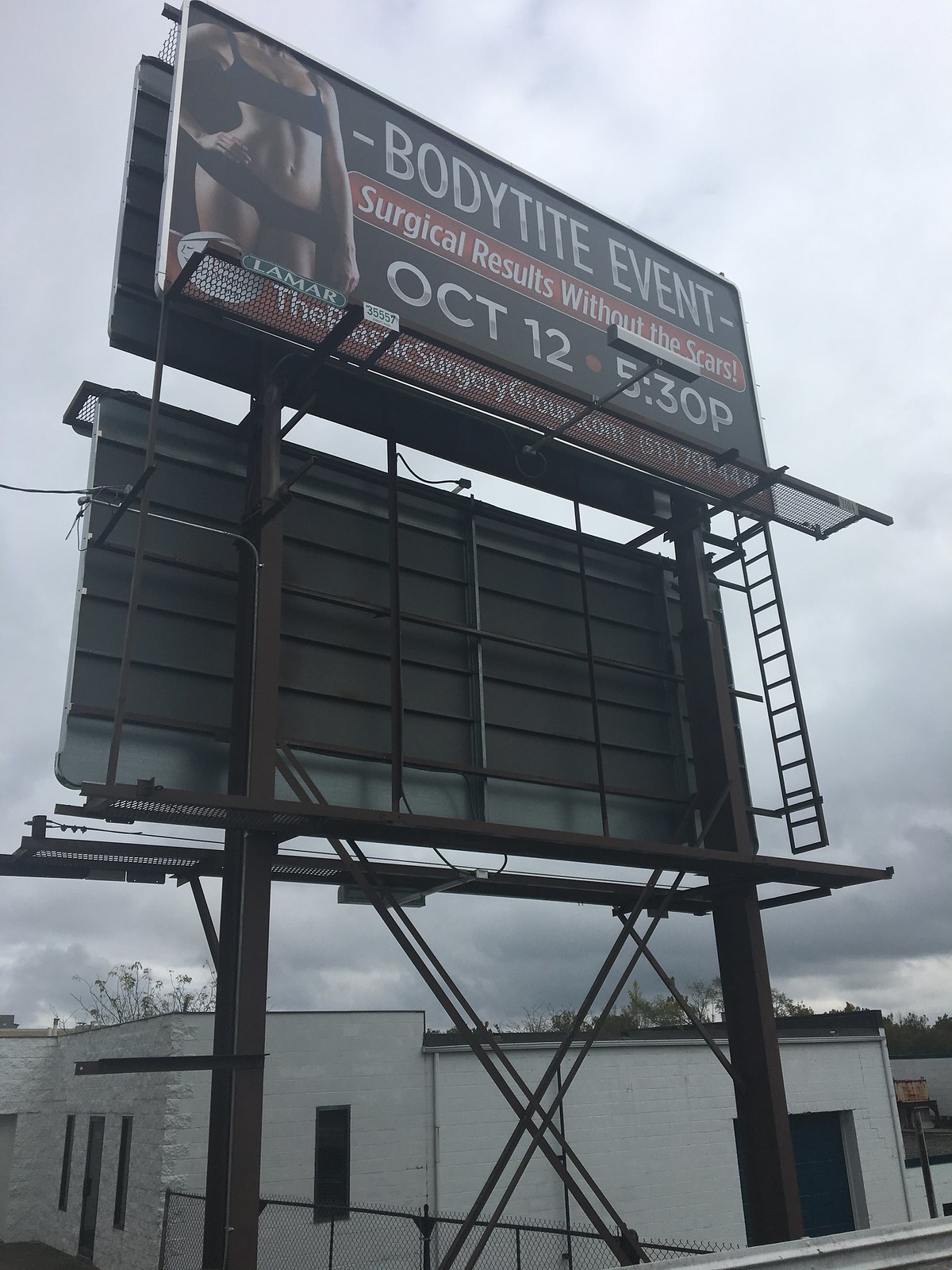The image depicts a cloudy, gray sky looming over a white building with black windows and a wide black door positioned to the right. In the foreground, a dark gray metal fence is lined below the building, with grayish-brown metal railings rising upward. Dominating the scene is a large outdoor billboard, supported by two substantial brown poles. The billboard features a woman dressed in a black sports bra and panties. The main sign reads "BODY TITE EVENT" in white letters against a black background, and highlights the event’s promise with a red banner stating "Surgical Results Without the Scars." Below this, it advertises the event date, "October 12th, 5:30 PM," in white lettering. The lower portion of the sign includes a gray banner with the word "Lamar" and a red section displaying "ThePlasticSurgeryGroup.com" alongside a phone number. Additional structural details include metal stairs ascending to the billboard, and the partial back view of another billboard situated behind the main one, secured by crisscrossing and downwards-supporting metal bars.